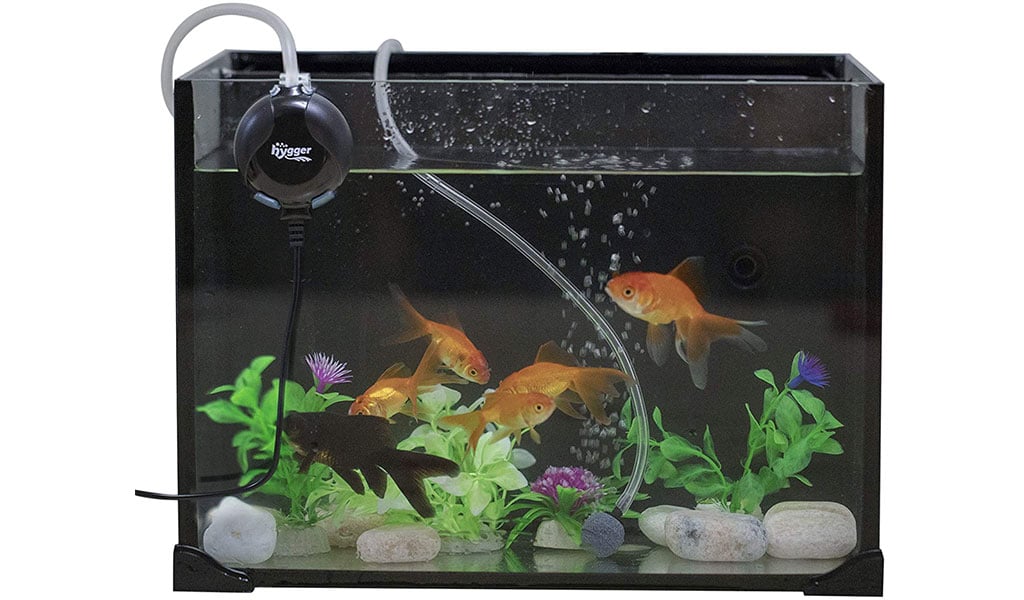A small, five-gallon aquarium is depicted, with a black border along three sides and a clear glass front. The tank houses about five goldfish, all displaying the typical orange and gold hues with some having fancy tails. They are somewhat clustered in the middle of the tank. The bottom of the aquarium features big rocks used to anchor a variety of fake plants, including green ones along with some adorned with purple and blue flowers. A black and white stone arrangement is also present. A filtration system is visible, featuring a clear tube that extends from a pump labelled "Higer" in white text on a black background, presumably connected to a power source outside the tank. The whole setup appears against a stark white backdrop, almost like a product image for a website. Bubbles can be seen rising to the surface, adding life to the contained aquatic scene.